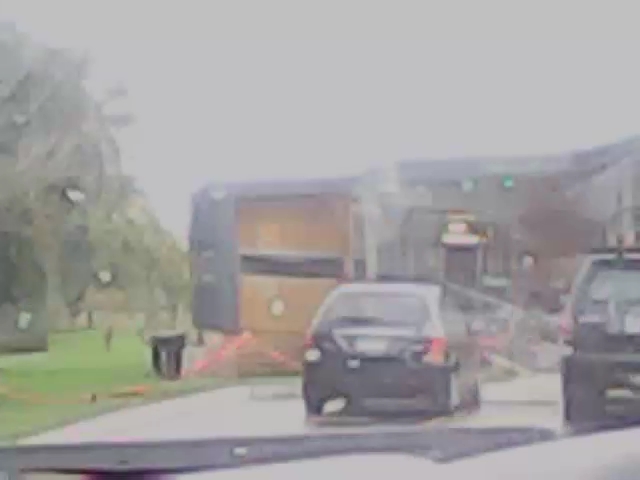A blurry daytime photograph taken through a rain-speckled windshield, showing a dashboard view of a road. There are a few cars ahead, including a black sedan in the center and a small black SUV partially visible to the right. The roadway is flanked by a grassy field on the left, with thick, gray clouds looming overhead. A red hose snakes through the grassy field, connecting a wooden building with a long horizontal window to both the front of the field and the right. Beside the building, on the left, there is a large residential trash can. The overall scene is wrapped in a fuzzy haze, giving it a dreamlike quality.